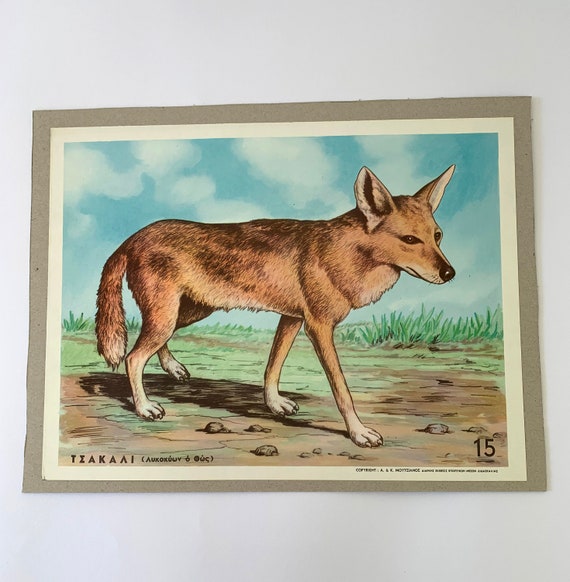The image showcases a detailed painting hanging on a white wall, prominently centered. The artwork features a dog-like creature, possibly a coyote or a wolf, characterized by its lean build, pointy ears, and black nose. The animal's coat is a mix of light brown to dark brown, with cream-colored paws. It is depicted walking from the left to the right side of the painting, its bushy tail hanging downwards.

The background consists of a dirt ground interspersed with small pebbles and short green grasses. Above, the sky transitions from a light blue to white, with smudges of clouds adding to the tranquil scene. 

The painting is bordered by a light brown outer edge and a cream-colored inner frame. At the bottom, there is a block of text reading "T-I-A-K-A-A" along with some smaller, less legible text, and the number "15" is distinctly noted in black in the bottom right corner.